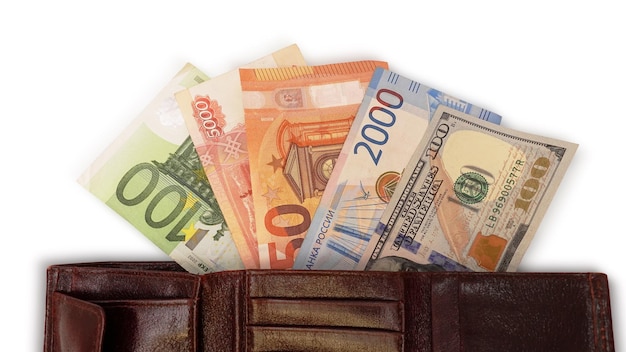The image features a brown leather foldover wallet set against a white background. The horizontally oriented photo showcases a variety of currency bills emerging from the wallet, indicating an international assortment. Prominently displayed are an American $100 bill, a Russian 2,000-ruble bill, and additional denominations including $50 and $5,000 bills from unspecified origins. The wallet itself is completely unfolded, revealing several small pouches, which are empty and devoid of any cards. This detailed scene captures the essence of global financial diversity.